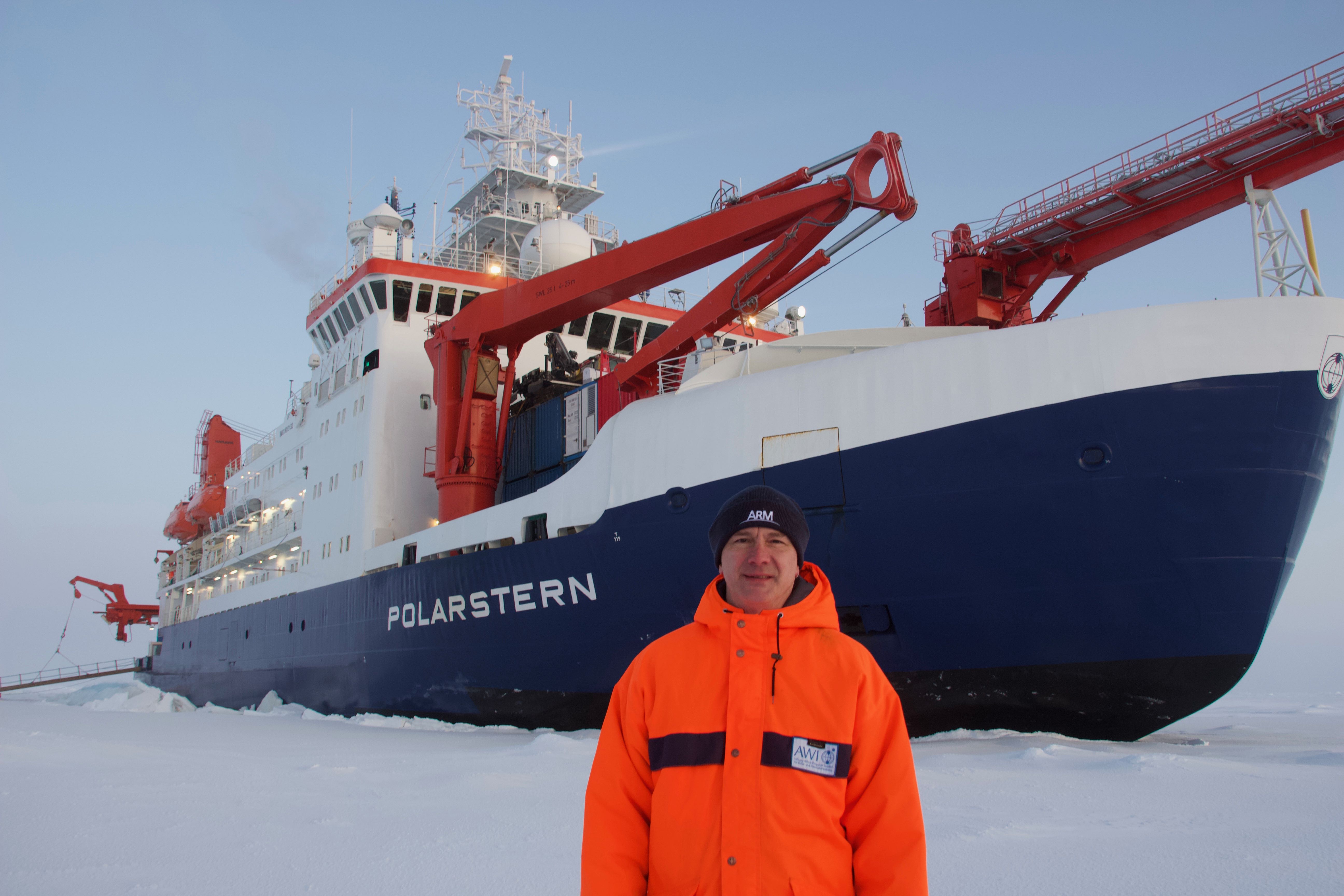In this captivating image, a large vessel named "Polar Stern," an icebreaker or coast guard ship, takes center stage. The ship, with a robust navy blue hull adorned with its name in bold white capital letters, is seemingly nestled amidst a snowy landscape, likely frozen in the icy water. The upper structure of the ship transitions to white, accented by prominent, reddish-orange cranes at the bow, extending towards the vessel’s midsection. An imposing command center with a tall, pointed structure, highlighted with red stripes, dominates the top, while additional cranes and lighting apparatus can be seen towards the aft.

Standing in the foreground is a man clad in a bright orange winter coat that is fully buttoned, featuring a black stripe with the letters "AWI." He also sports a black stocking cap emblazoned with "ARM" in white letters. The clear, light blue sky and his cheery, smiling demeanor suggest a brisk but clear day, capturing the quiet majesty of the frozen, remote setting. This detailed composition blends the rugged resilience of the maritime vessel with the human spirit of exploration amid the stark, icy wilderness.